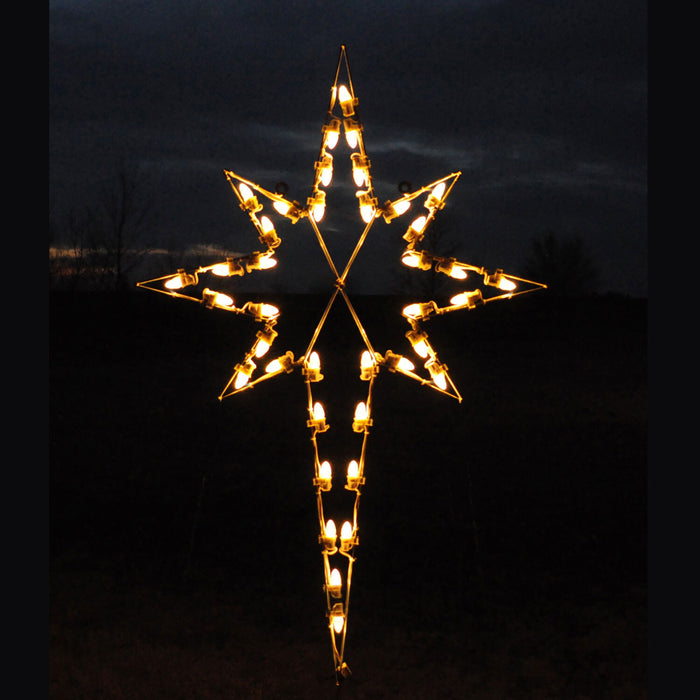The image depicts a nighttime scene with a dark sky and minimal illumination, primarily from moonlight and scattered white clouds in the upper portion of the picture. The background reveals the faint outlines of a town, with lights visible on the left side, while the right side is more obscured by darkness and trees, including a leafless tree on the left side. Dominating the center of the image is a lit-up Christmas star decoration. The star features a prominent, elongated bottom point extending from the middle, flanked by three points on each side, with the central side points being longer than the adjacent ones. The top point of the star is slightly shorter than the bottom point but longer than the side points. The star is illuminated with yellow-white lights and appears suitable for outdoor decoration, possibly on a tree, deck, or fence.